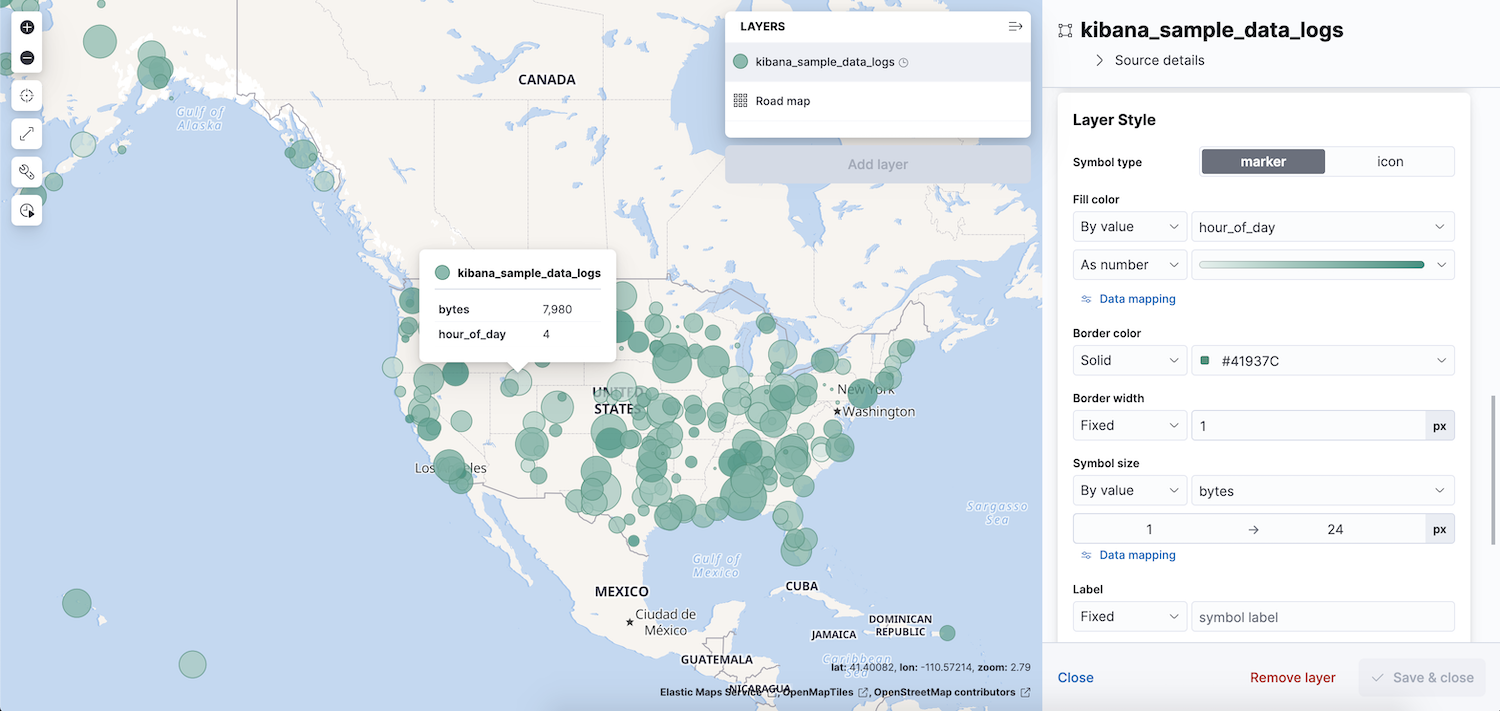A detailed and cleaned-up caption for the described image could be:

"A computer screen capture displays a demographic map focusing on data usage patterns across North America, including parts of Canada, the United States, Mexico, and some Central American countries. The map is overlaid with multiple gray road maps and green circles of varying sizes, representing different concentrations of data activity. The title 'Cabana Sample Data Logs' is prominently featured, indicating that the data might be related to some form of consumption or search activity, possibly matched to certain times of the day. A noteworthy data point shows a circle labeled with '7,000+ bytes per hour,' suggesting intensive data usage. On the right-hand side of the screen, there are various layer style symbols and markers used to differentiate information by color and time of day. Although the exact nature of the data is unclear, the visual elements suggest a complex analysis of demographic data usage trends."